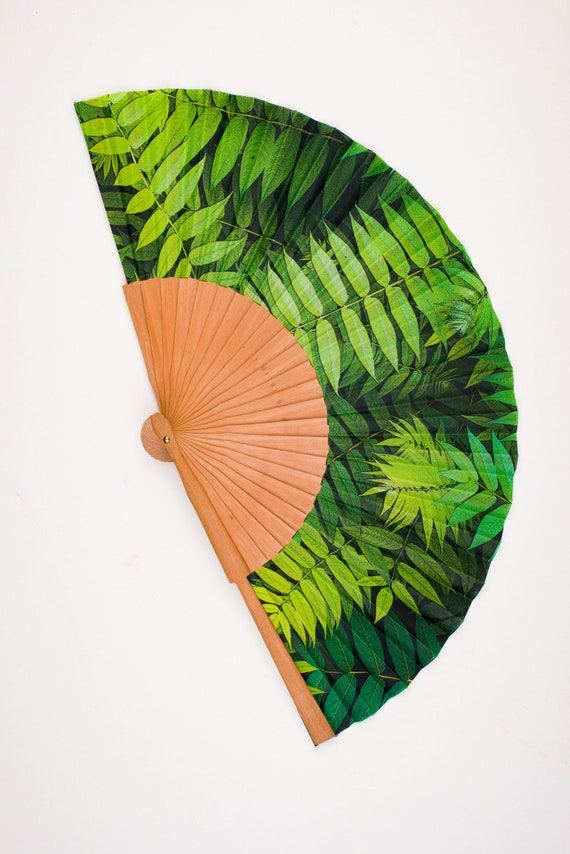This is a detailed photograph of a traditional Japanese-style hand fan, fully opened in a semi-circle and placed on a neutral beige background. The fan features an intricate design on the outer portion, showcasing various shades of spring medium to dark green leaves, resembling ferns or perhaps forest tree leaves. The leaves create a vibrant, canopy-like effect against a black patterned background. The inner portion of the fan is made of light blonde wood, with visible wooden spines that support the structure. The handle, also wooden, is simple and unadorned. There are no signatures, logos, or additional markings on the fan, enhancing its minimalist yet colorful appearance.